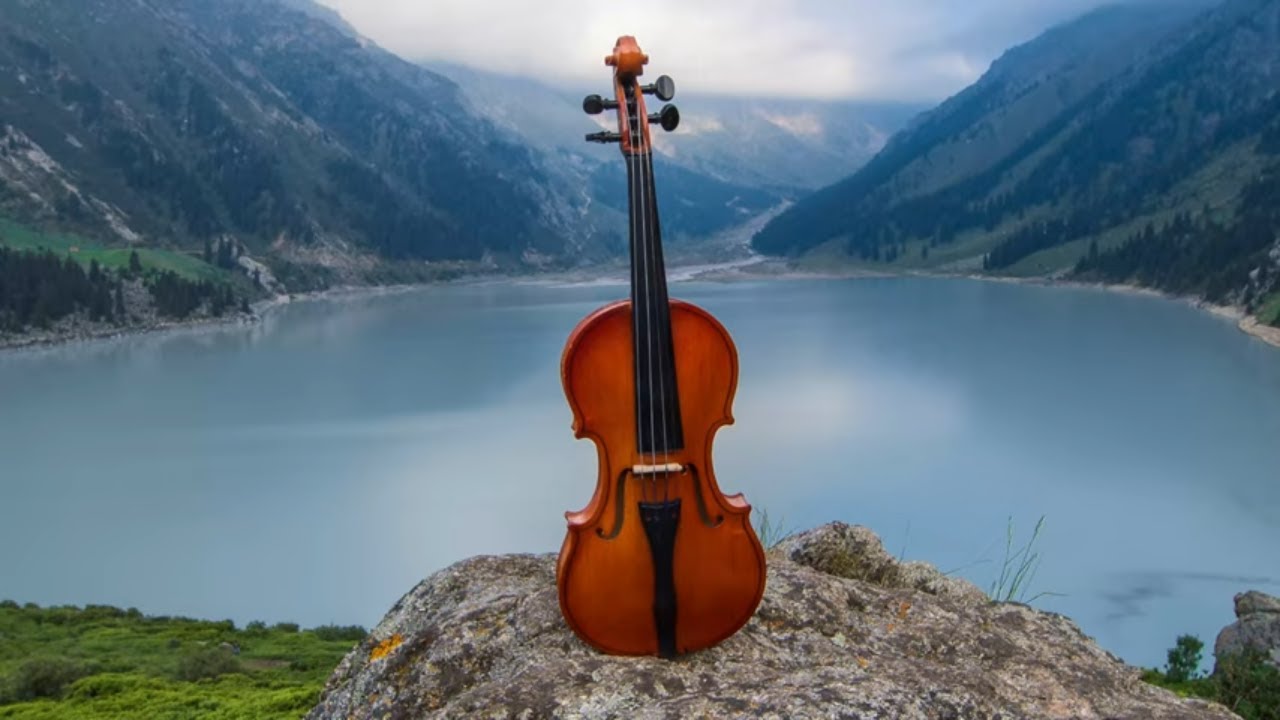This vibrant full-color photograph, clearly staged and captured outdoors during the day using natural light, offers an awe-inspiring view. The vertically rectangular image has no border or specific background, featuring a serene natural setting. At the top middle of the photograph, a cloudy and overcast sky is depicted, flanked by majestic mountains on each side. These mountains, abundant with evergreen vegetation, gently slope upwards, while far in the distance, additional mountains create a hazy backdrop.

Dominating the center of the image is a calm and reflective lake, its surface so still that it mirrors the clouds above. The lake's tranquil, grayish-blue water enhances the peaceful atmosphere. Along the lower left and right edges of the photograph, patches of vibrant green grass add a touch of lushness to the scene. 

In the foreground, centrally positioned, is a large gray rock. Perched atop this rock is a beautifully crafted wooden violin, standing upright without any visible support. The violin's rich brown hue contrasts with the rock and surrounding landscape, making it the focal point of this meticulously composed scene. There are no people, text, or watermarks in the image, allowing the viewer to fully absorb the natural beauty and artistic arrangement of the violin in this mountain setting.